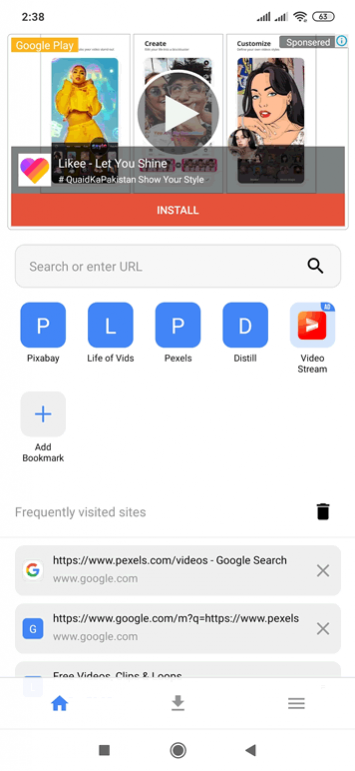The image appears to be a screenshot of a smartphone’s browsing activity and interface. At the top, there is a prominent ad banner for the Google Play Store featuring various visuals: a woman dressed in yellow, two individuals posing for the camera, and a cartoonish depiction of a woman. The ad text reads “Likee: Let You Shine #quadK Pakistan Show Your Style” with a red "Install" button underneath.

Below the ad, there is a search bar with the placeholder text “Search or enter URL.” Directly under the search bar, several bookmarks are displayed as thumbnails labeled: "Pixabay," "Life of Vids," "Pexels," and "Distill Video Stream," along with an additional thumbnail labeled "Add Bookmark."

Underneath the bookmarks, a section labeled "Frequently Visited Sites" is visible, containing a small trash can icon next to the entries "pexels.com" and "google.com." There is also partial text visible that reads "Free videos clips and loops," which is cut off by interface elements at the bottom of the screen.

At the bottom of the image is the smartphone’s navigation bar, showing icons including a house symbol for the home screen, a download icon, and three horizontal lines likely representing a menu. Centrally located are navigation controls: a square on the left, a circle in the center, and a left-pointing arrow on the right.